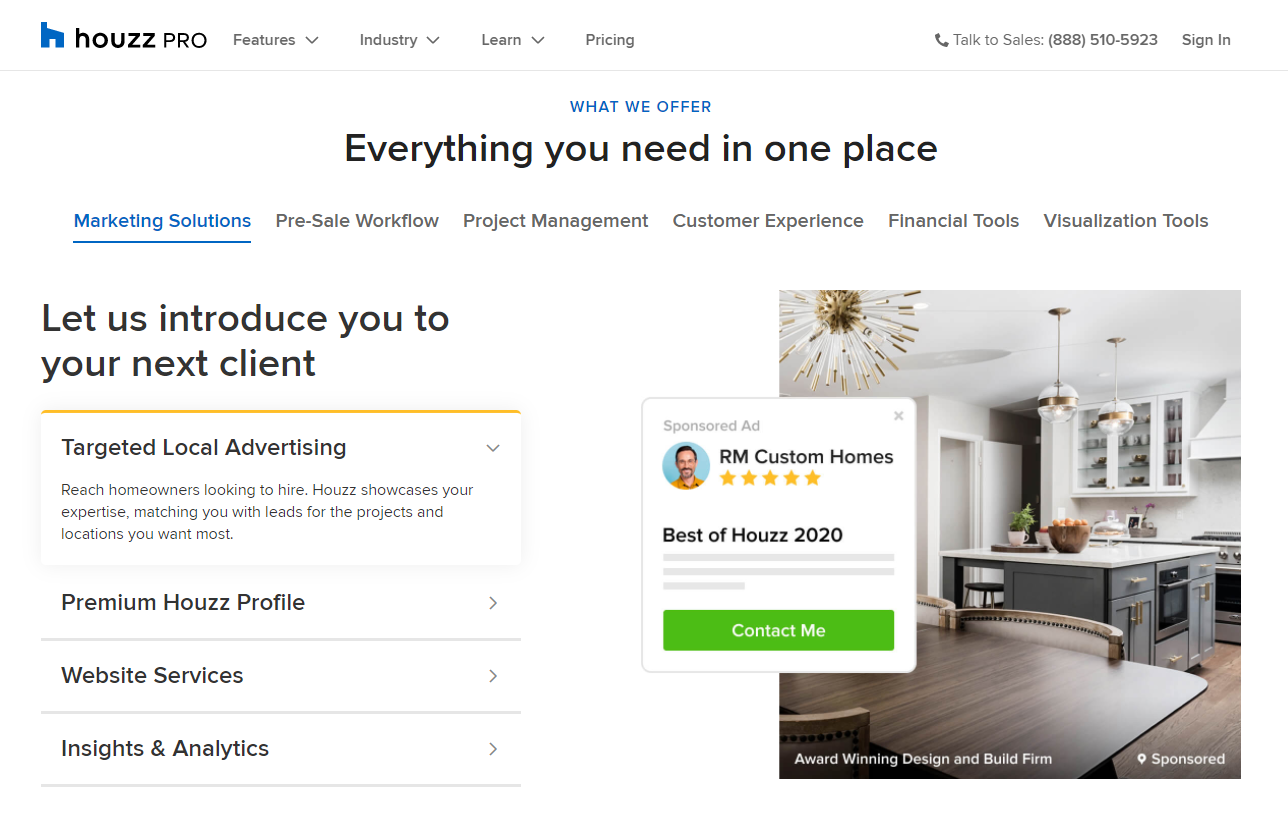A detailed caption for the image could be:

"This image showcases the homepage of a website called House Pro, which appears to specialize in real estate services. At the top, there is a distinctive blue house-shaped icon with the site's name, 'Houzz Pro,' followed by navigation menus labeled 'Features,' 'Industry,' 'Learn,' and 'Pricing.' The header also includes a contact phone number. Below this, a bold slogan reads, 'Everything you need in one place,' emphasizing the site's comprehensive offerings, which range from marketing solutions and pre-sale workflows to project management, customer experience, financial tools, and visualization tools. The section promises to introduce users to their next client with targeted local advertising, premium house profiles, website services, insights, and analytics. 

The focal point of the image is a modern kitchen, featuring sleek white counters, gray cabinetry, a white glass wine holder, and pristine white walls, encapsulating a contemporary design aesthetic. Overlapping the bottom right section of the kitchen image is a pop-up ad for RM Custom Homes, touting a 'Best of Houzz 2020' award with a five-star rating, including a prompt to 'Contact me.'"